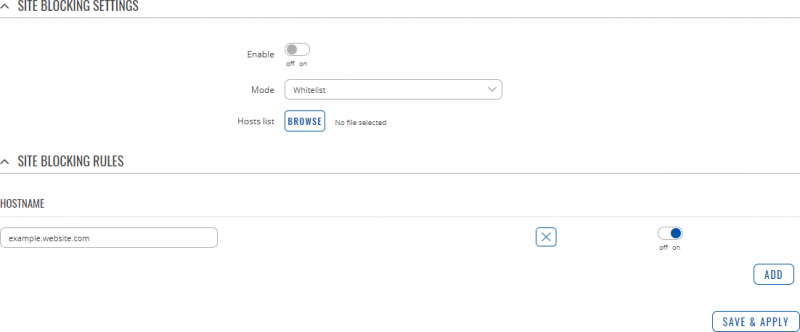Screenshot of a Site Blocking Settings Page on an Unknown Website

The screenshot captures a site blocking settings configuration page of an unidentified website. The interface is displayed on a white background with black and gray text, and some interactive elements in blue.

- The top section of the page contains the title "Site Blocking Settings," flanked by options to "Enable" the feature with choices "Off" or "On." The slider switch for enabling site blocking is toggled to "Off."
- Below this section, options for selecting the blocking mode are shown, labeled "Mode, White List, Hosts List." Next to this is a button labeled "Browse," with the adjacent text indicating "No File Selected."
- Further down, there is a section titled "Site Blocking Rules," which includes a search bar containing the example entry "example.website.com." To the far right of this input field is a blue "X" inside a blue square for deletion of the entry.
- Beneath the search bar, another slider button allows toggling between "Off" and "On," with the button selected to "On."
- At the bottom of the interface, there are options to "Add," "Save," and "Apply" changes, all highlighted in blue.

The image is notably text-heavy and lacks any illustrative or photographic elements. It consists purely of navigational and user interface elements without any depiction of people, animals, plants, buildings, birds, fish, or bicycles. The format of the image is much wider than it is tall.